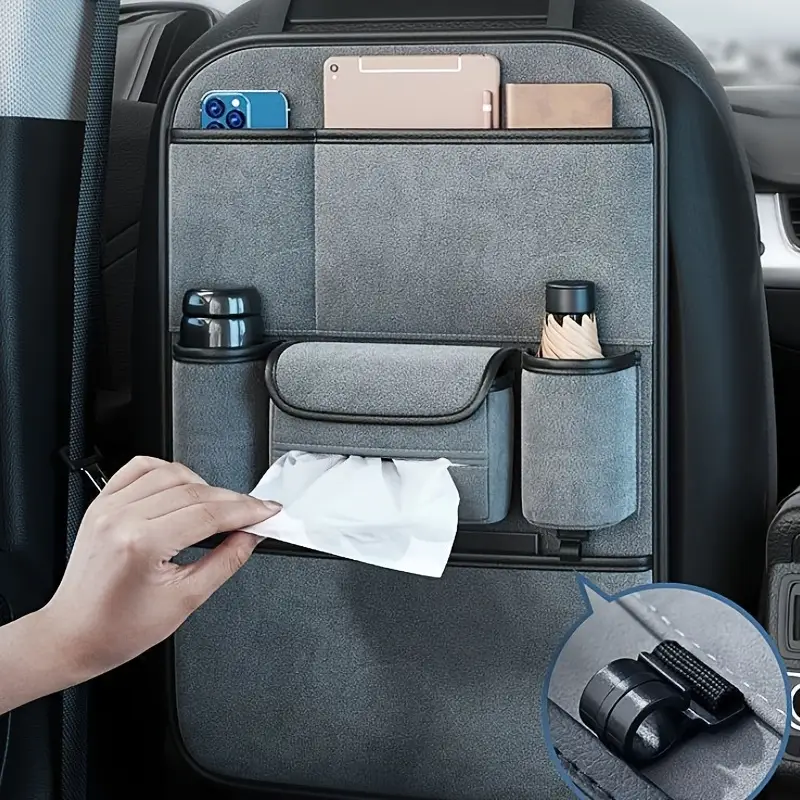The photograph captures the back of the driver’s seat inside a vehicle, showcasing a detailed and well-organized multi-pocket storage system made from light gray suede with dark gray or black vinyl borders. The organizer features three tiers of storage. The top tier has two pockets: the left one holding a small blue smartphone and the right one containing a light rose pink iPad with an attached stylus and a wallet. Below these, the second tier consists of two cup holders; the left one is occupied by a black thermos, and the right one holds either a black bottle or a folded umbrella. Between these cup holders is an oblong compartment with a flap covering a tissue dispenser, from which a piece of tissue is being pulled by a Caucasian hand entering from the left side of the image. The bottom of the organizer has an additional large pocket whose contents are not visible. In the bottom right corner of the image, an inset highlights a close-up of a small black clip designed to secure the umbrella holder to the organizer.